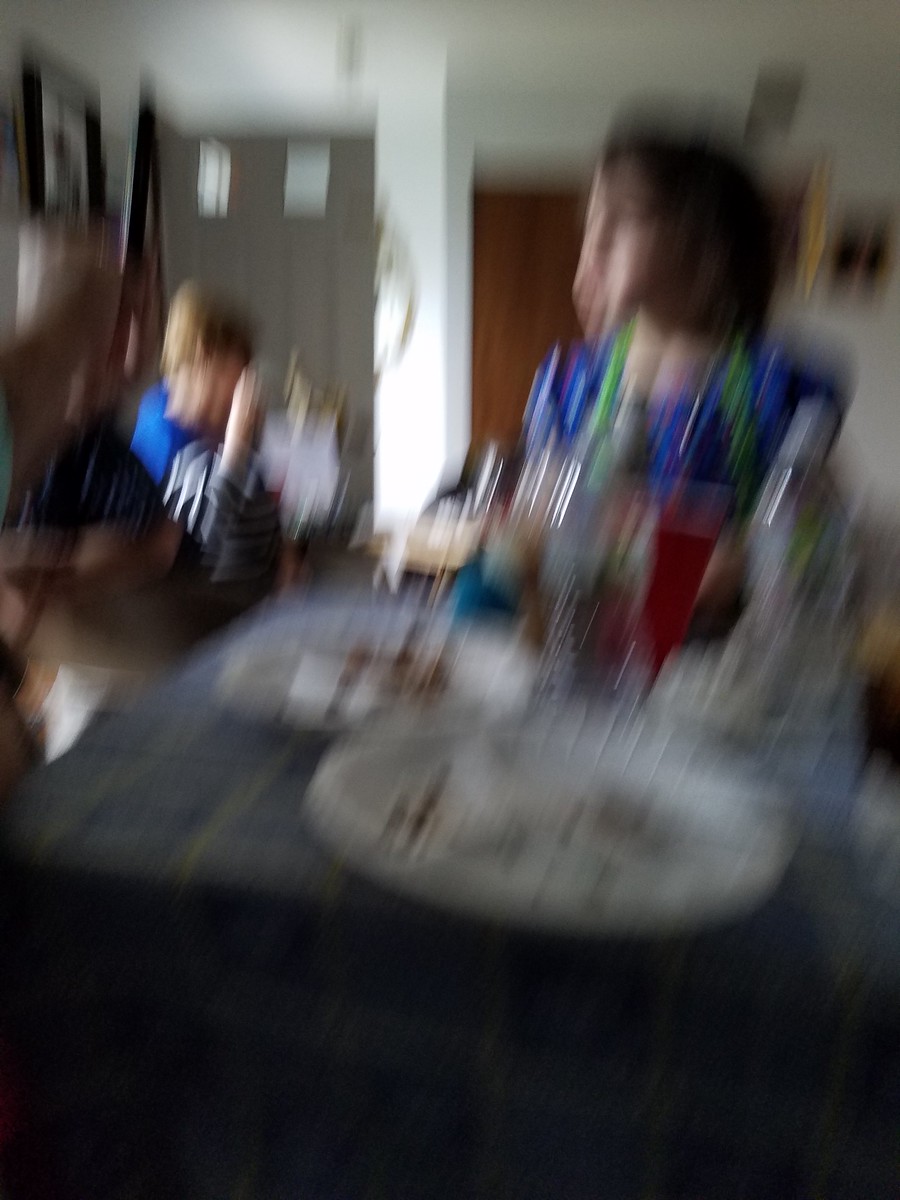A very blurry photograph appears to capture a domestic scene inside a home. In the foreground, a child can be discerned, though without sharp clarity, and behind them, there might be a parent or possibly another child. The far background of the image hints at a door, while in the immediate foreground, two plates are resting on what might be either a couch cushion or a table adorned with a plaid tablecloth. The efforts to take the photo resulted in much blur, making details hard to pinpoint. Natural daylight filters in, likely from a nearby window, giving the scene a soft, ambient light without the sharpness of a flash. On the plates and the surface before them are some indistinguishable items, and there seems to be a glass containing a red liquid, adding a touch of color to the otherwise hazy tableau.